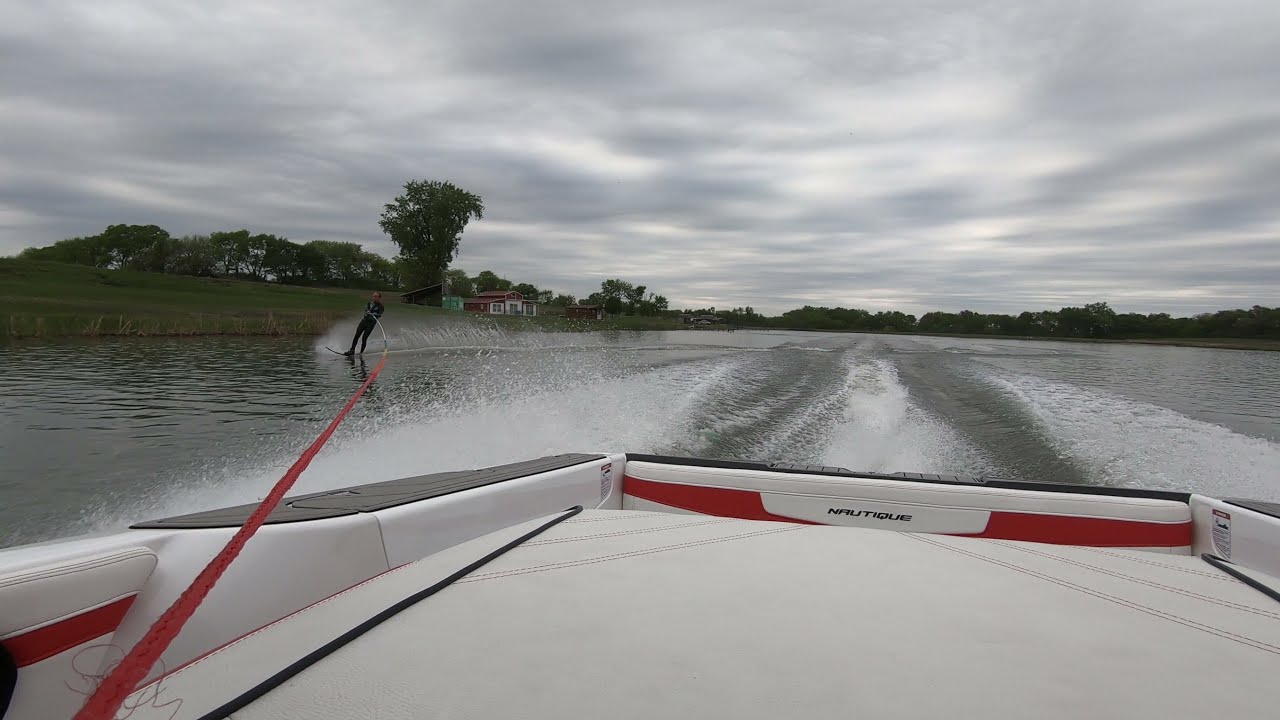The photograph captures an action-packed scene from the back of a speeding Nautique speedboat, which is white with red accents. The boat features a protective white cover at the rear to shield it from splashing water. The powerful motor, positioned below, churns up significant wakes on either side, with white spray rising dramatically. A red rope extends from the boat to the water skier, who is gliding on the surface, having just crossed the boat's wake to the right side of the frame. The skier, dressed in a black outfit and positioned on the left side relative to the boat's centerline, is about 20-30 feet from the grassy shore, which is lined with trees and possibly some distant cabins. The water appears gray and turbulent, indicating the boat's fast pace. Overhead, the sky is cloudy and overcast, adding a cooler, perhaps brisk atmosphere to the scene.